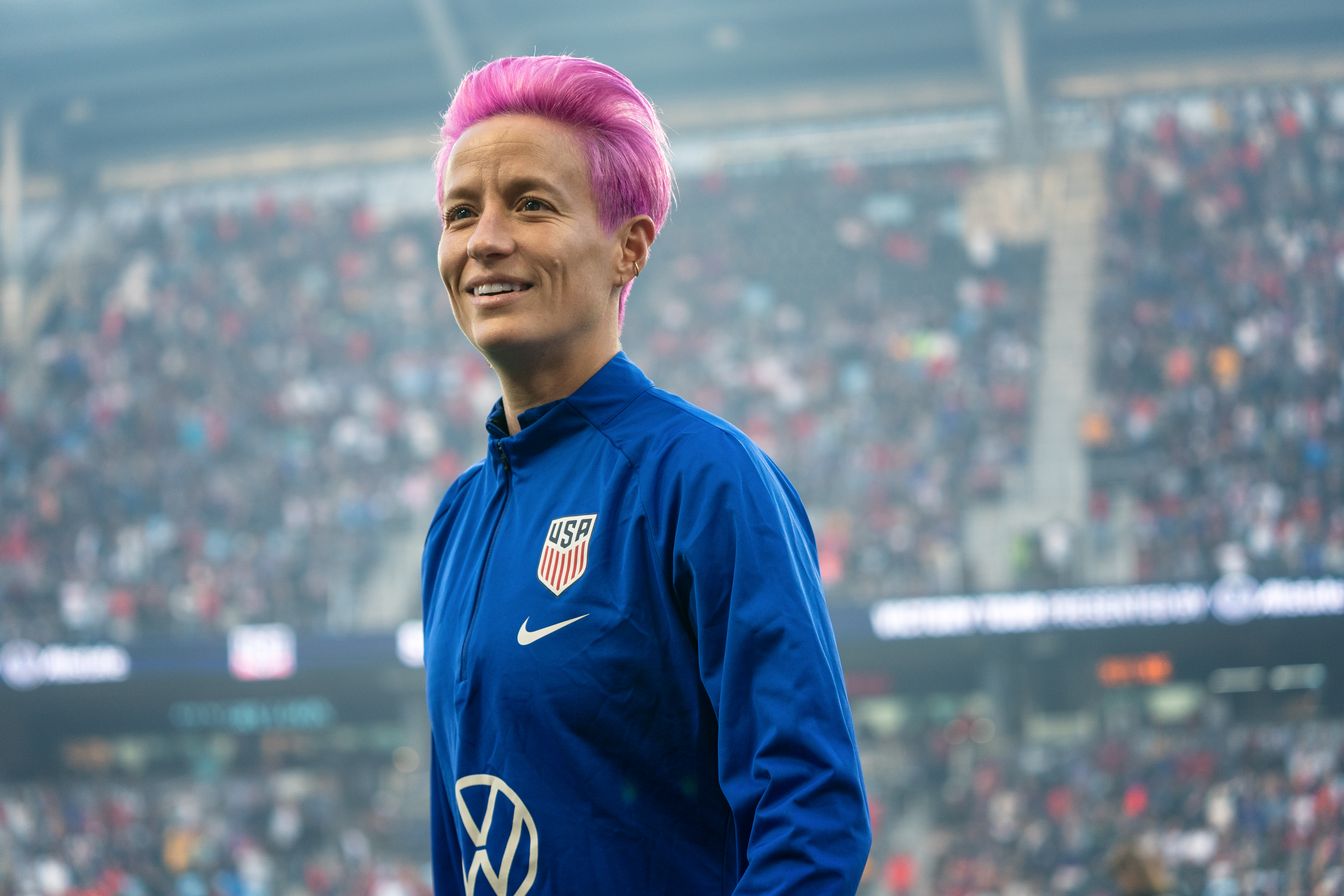This is a detailed photograph of Megan Rapinoe, a well-known FIFA soccer player, standing in a large, packed stadium. The venue features two levels of seating, both completely filled with enthusiastic fans. The stadium has an extensive awning or roof coverage, especially noticeable over the higher, steeply-angled seats. 

Megan Rapinoe, centrally positioned in the image, wears a blue jacket adorned with a Nike logo, a USA badge with red stripes representing the United States flag, and a VW logo on her chest. She has distinct short pink hair and a fair complexion. Her gaze is directed to the left, capturing a moment of focus and intensity amidst the lively atmosphere of the arena.